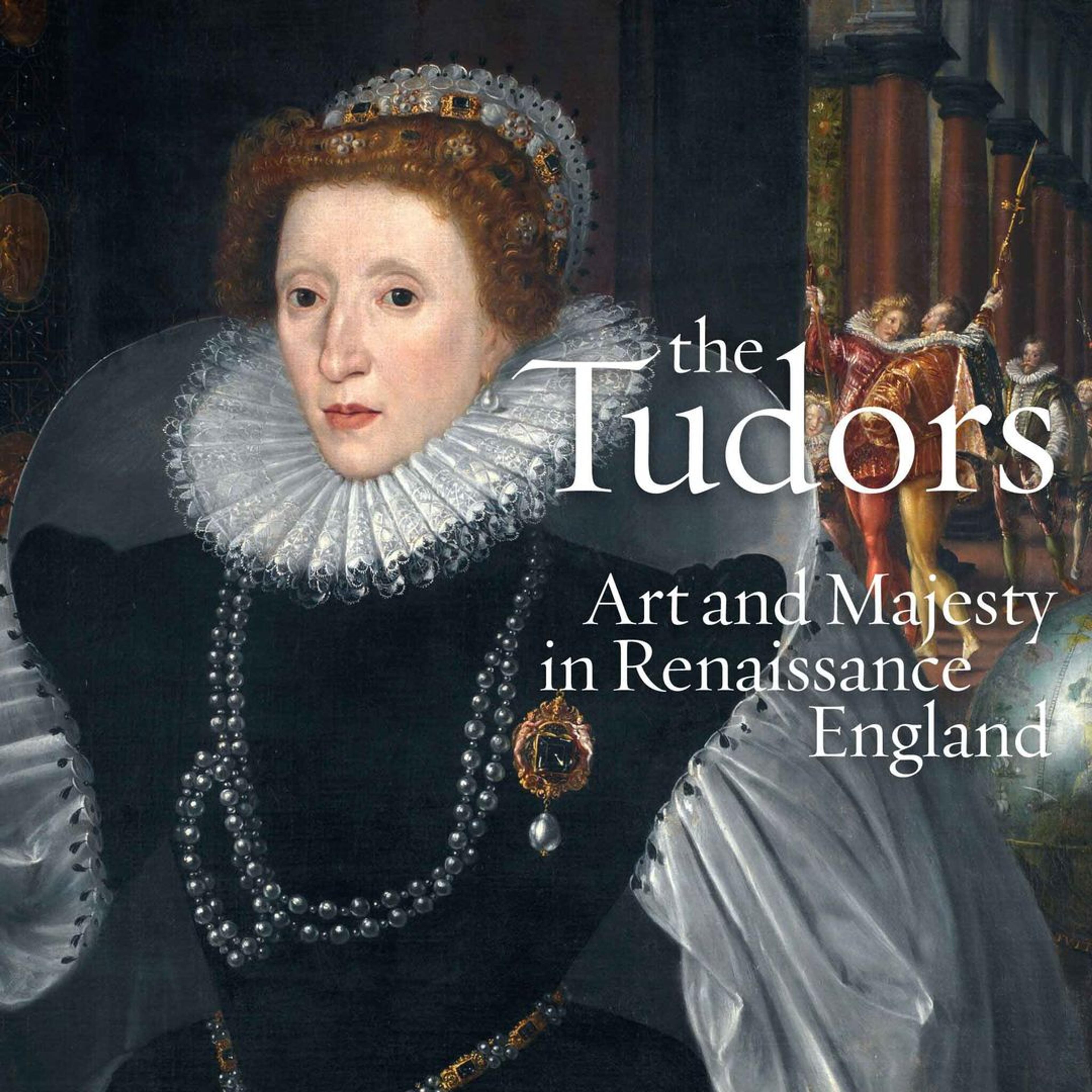This image depicts a regal painting of Queen Elizabeth I, characterized by her austere expression and detailed Renaissance attire. Her red hair is styled back, with a portion visible, adorned with a headdress accented by gold stones. Her dark brown eyes and pale red lips add to her stoic demeanor. The Queen is garbed in a striking dress that is predominantly black or navy, with elaborate puffy sleeves that are light gray. A large, ornate white collar encircles her neck, from which hangs silver beads and a prominent brooch resembling a yellow flower with a pearl extending down from it. Around her waist, jewels embellish her cinched silhouette, complemented by a string of gray pearls. 

In the background, a scene featuring courtiers, both men and women dressed in attire indicative of the era, appears to show them engaged in a heated discussion or conflict. The image is overlaid with text: "The Tudors" in large white letters, with "Art and Majesty in Renaissance England" written beneath it in slightly smaller white text, suggesting that this image could be from a book or an album cover celebrating Tudor art and majesty.